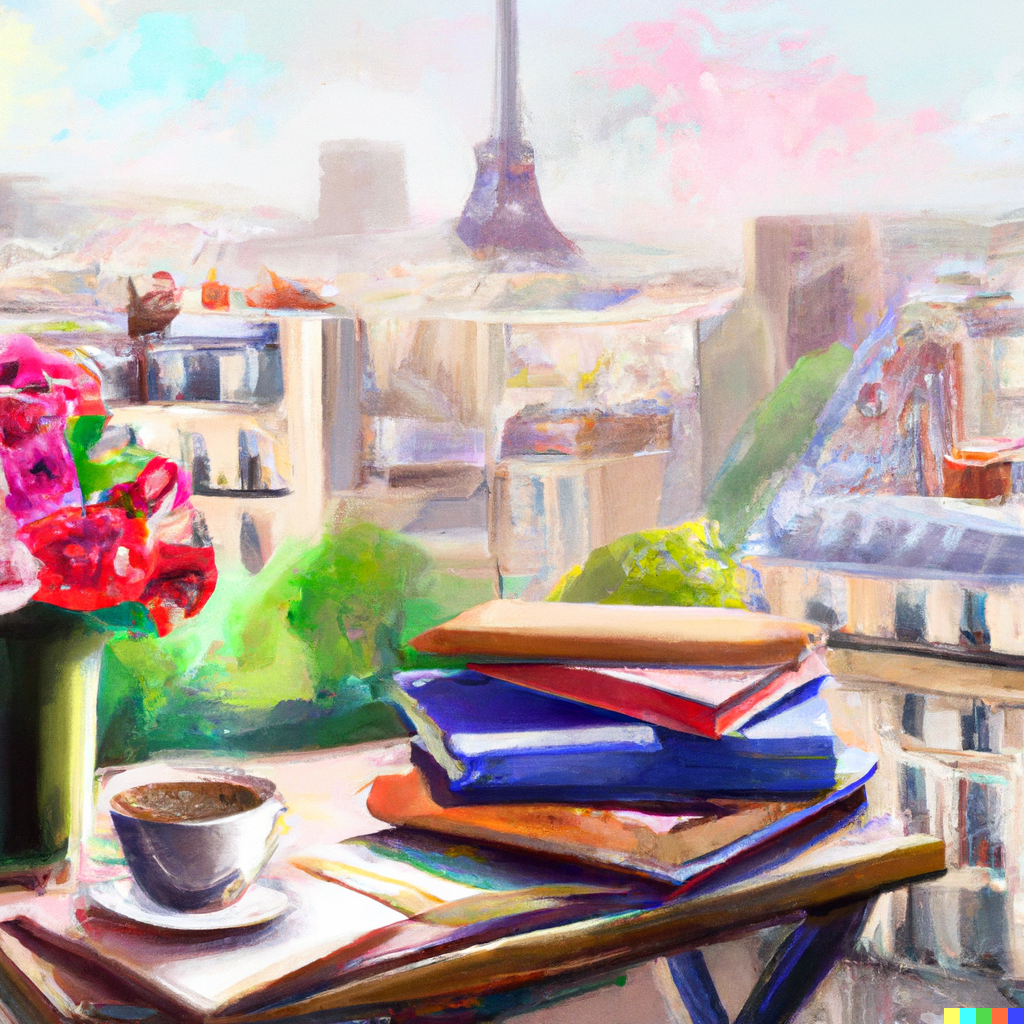The watercolor painting depicts a vibrant Parisian scene viewed from a balcony. The centerpiece of the background is the iconic Eiffel Tower, with its distinctive blue base rising into a thin spire, surrounded by foggy gray. To the left of the Eiffel Tower stands another tall building. The right side of the canvas showcases a cluster of soft pink clouds. Below the skyline are light brown rectangular buildings interspersed with green trees. In the foreground sits a rectangular, slightly tilted wooden table adorned with four stacked books colored orange, blue, red, and light brown. To the left side of the table, a green vase overflows with red and pink flowers, complemented by a coffee cup filled with black coffee. This charming tableau captures an essence of chic Parisian lifestyle, blending urban elements with cozy details.